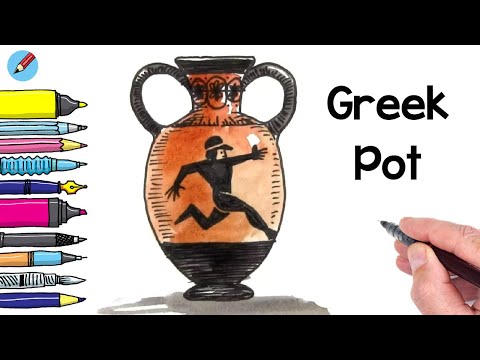The image appears to be a digitally illustrated instructional design, possibly a header for a website or a thumbnail for a YouTube video. It features solid black bars across the top and bottom, each taking up about an eighth of the page. On the left side, a blue square with a red pencil tip that says "easy" serves as a logo. Below the logo, the blue handwriting-style text reads, "draw an ancient Greek pot."

Occupying the right half of the image is a detailed drawing of an ancient Greek pot. The pot has a small neck, two black handles extending from the neck to the body, and is predominantly tan with black accents. The base, handles, and rim of the pot are black, and it has a circular pattern near the top. The pot’s body features an image of a muscular, athletic man dressed entirely in black, depicted mid-stride as if running. The entire pot has a glossy, glazed appearance, suggesting a realistic and polished finish.